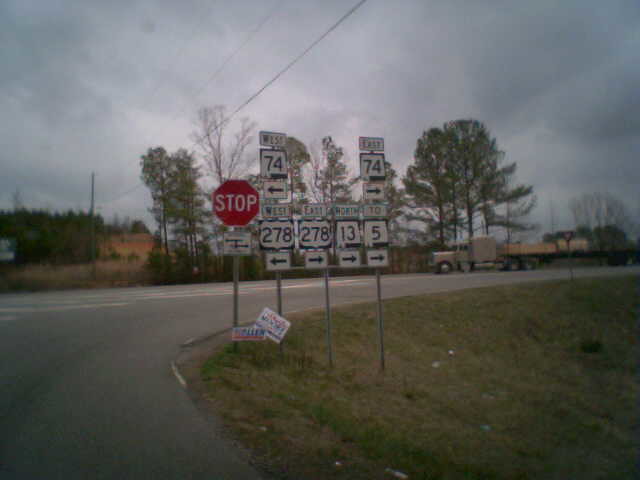A vibrant outdoor scene featuring an intersection crowded with various directional signs. Dominating the foreground is a prominent red stop sign, beneath which are several political campaign signs. To the right of the stop sign, a series of directional signs guide travelers: a "West 74" sign with a left arrow, a "West 278" sign also pointing left, an "East 278" sign with a right arrow, a "North 13" sign pointing right, an "East 74" sign directing right, and finally, a "252 and 5" sign pointing right as well. Trees form a lush green backdrop, adding a splash of natural color to the scene. On the far right, a truck is visible, completing this bustling roadside snapshot.